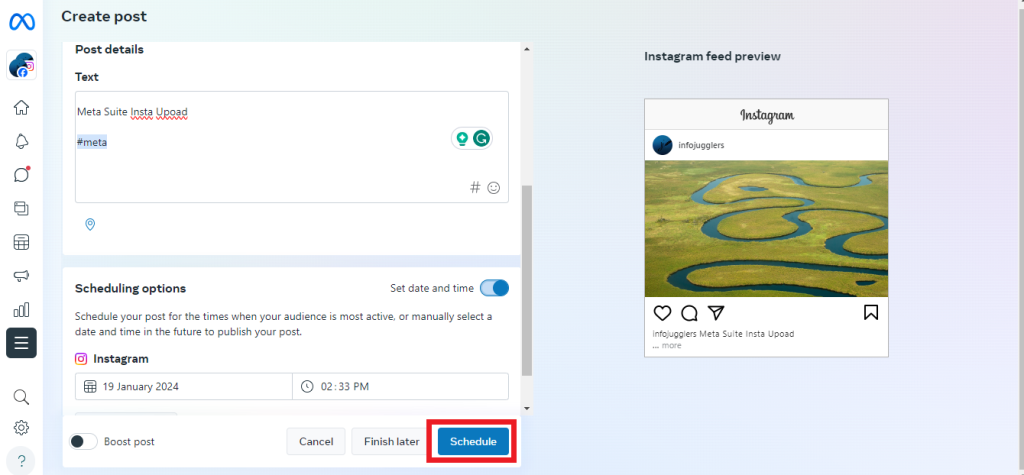The image is a detailed screenshot from a Meta interface. On the left-hand side, a white background extends from the top left corner to the bottom left corner, displaying various options including accounts, homepage, notifications, messages, tabs, groups, calendar, settings, a search bar, and a menu button. 

To the right, the background transitions into a gradient ranging from light blue to light purple. Centered within this gradient, there is a white box where post details can be entered. The text box contains the input "meta suite insta up code," with a hashtag "#meta." Notably, the intended word "upload" is misspelled as "up code," missing the letter "L."

Beneath this text box, another white box shows scheduling options, where the user has toggled the ability to set the date and time for the post. The post is scheduled to be uploaded to Instagram on January 19th, 2024, at 2:33 PM. The schedule button is prominently displayed in blue with white text, outlined in red to draw attention.

Additionally, on the right-hand side of the image, an Instagram feed preview is visible, showing a mock-up of the user's post as it will appear once uploaded.